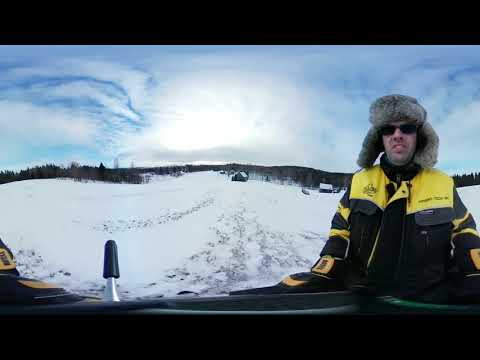In this outdoor winter scene, a man stands prominently in the right foreground. He appears to be of Caucasian ethnicity, wearing a fur-lined hat, black sunglasses, and a heavy black parka with a yellow collar and yellow stripes on the sleeves, giving him a somewhat frowny appearance. The ground is covered with snow, presenting a wintry landscape. Directly in front of him is a complex contraption, possibly a vehicle or conveyance, featuring a black handle on a red, silver, and white metal frame fixed to a bar. The scene is set against a cloudy blue sky, with the bright white sun partially obscured by thin clouds. The horizon, visible in the middle ground, is irregular, dotted with spiky trees. In the distance, a tiny house can be seen, providing a solitary aspect to the otherwise expansive snowy terrain.